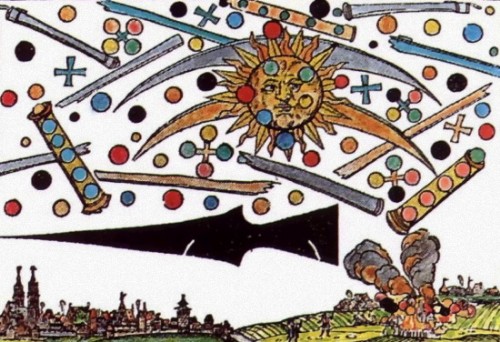A stylized drawing illustrates a vibrant cityscape under a whimsical sky. Dominating the foreground, the bottom right corner features detailed strips of yellow and green cultivated farmland. At its heart, a burning building emits dramatic red and black puffs of smoke, adding urgency and contrast to the serene agricultural scene. On the bottom left, a medieval cityscape emerges, characterized by numerous towers and two prominent spires that soar above the rest. The majority of the composition is occupied by a white sky, dominated by a large sun with a human face, beaming with yellow and orange rays. The sun's visage is adorned with colorful dots—red, yellow, blue, black, and green—that pepper the entire sky. Purple, black, and grey rods further fill the sky, creating a lively, almost chaotic backdrop that enhances the narrative complexity of the scene.